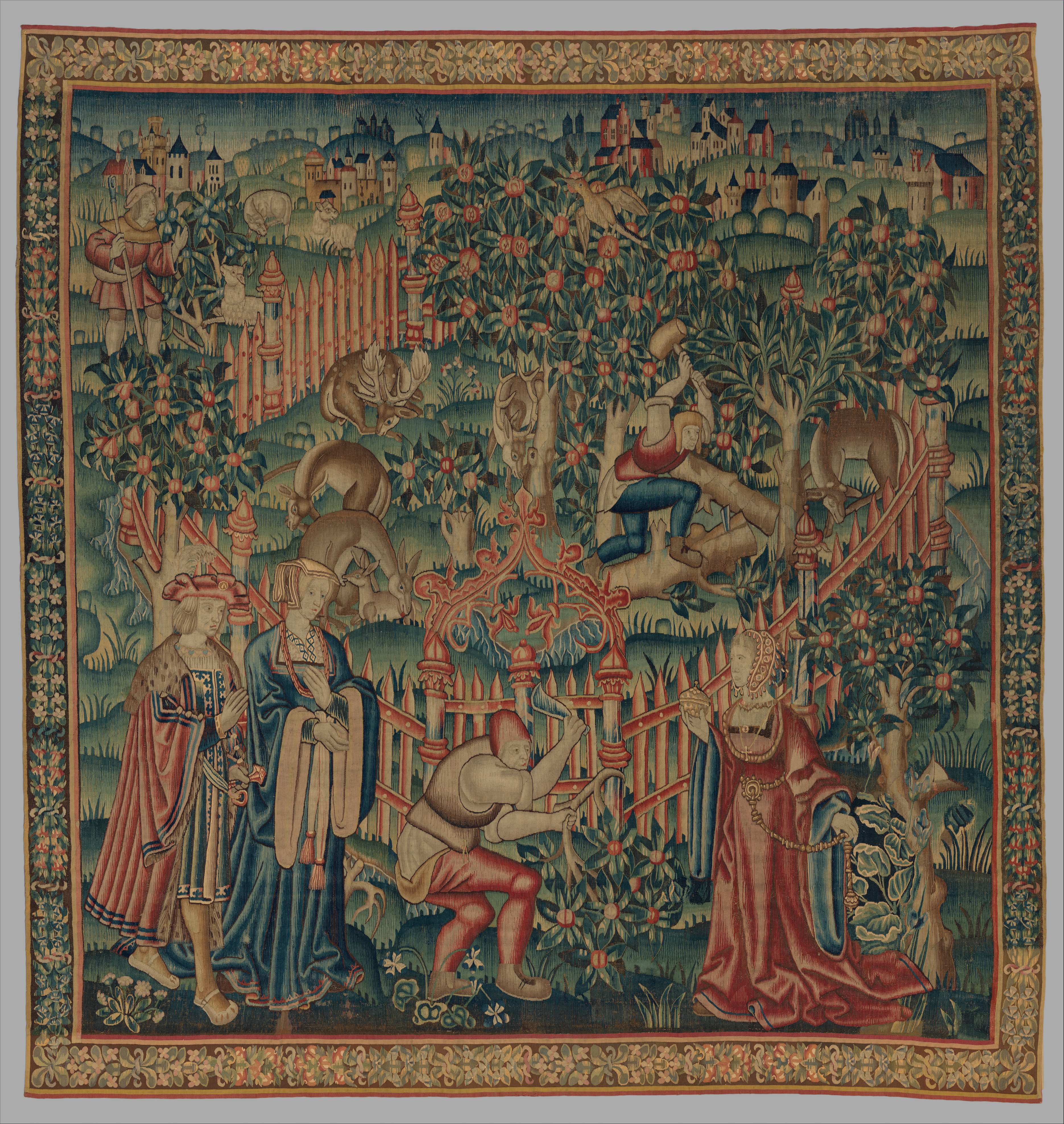This image appears to be an elaborate Renaissance tapestry, characterized by its subdued goldish hues blended with rich reds, greens, and blues. The foreground prominently features four figures. A young woman in a red dress, accented with blue interior, stands on the right side, looking thoughtfully to the left. Nearby, a man crouched as if preparing to throw something, possibly a jester, is depicted with striking detail. Behind him, another man adorned in a blue cape showcases large, muscular arms, while beside him, someone in a Robin Hood-style hat and red cape stands poised.

In the midsection, a fenced area, imbued with an orangish color, encloses a pastoral scene. Fruit trees, possibly bearing pears and peaches, dot the landscape, and a male figure, wielding an axe or hammer, appears to be splitting a tree. This area is also grazed by several deer, adding a touch of woodland serenity.

Further back, additional figures emerge; a man appears to offer a branch to the woman or perhaps is engaged in cutting it down. Another duo—potentially a man and a woman—stand by, overseeing the activities. Scattered throughout the background are medieval architectural elements, including castles and turrets, nestled among rolling hills, enhancing the scene's historical ambiance. Framing this intricate tableau is a subtle, monotone gray and white border, suggesting it might be hung on a wall, highlighting the tapestry's intricate craftsmanship and artistic detail.